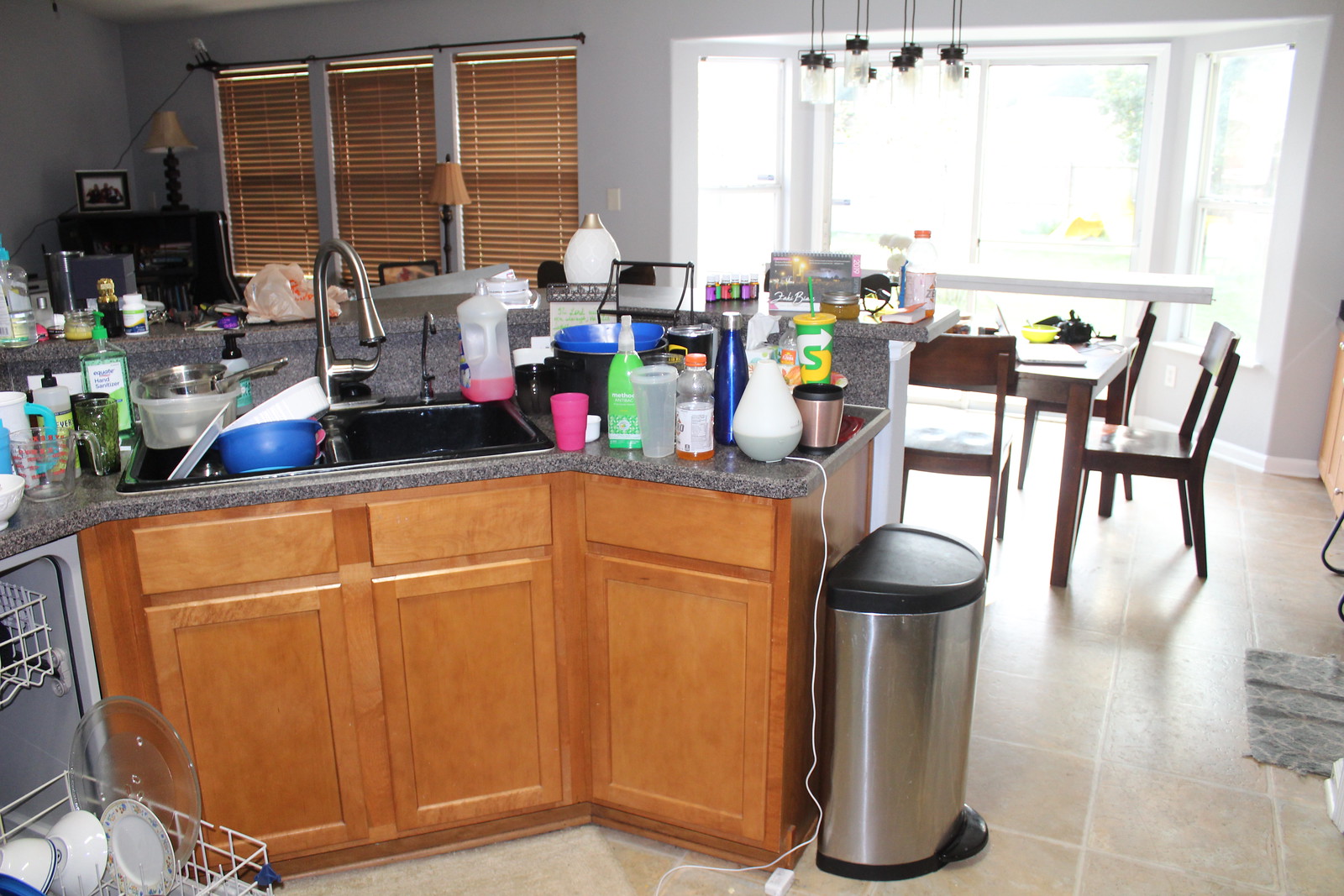This vivid color photograph captures a bustling kitchen scene. In the bottom left corner, an open dishwasher reveals numerous plates and bowls arranged in the extended bottom rack. The kitchen cabinets below and to the right of the sink are crafted from dark wood, imparting a rich, warm tone to the setting. The black granite countertop is densely cluttered with various items, including measuring cups, drinking glasses, hand soap, hand sanitizer, an oil diffuser, a blue metal reusable drinking bottle, a half-empty bottle of energy drink, and a Subway cup. The left side of the sink is filled with dirty dishes.

Behind the sink, a secondary counter is equally cluttered with items: plastic bags, vitamin bottles, candles, another oil diffuser, and what seems to be an assortment of nail polish bottles. In the background, a framed picture and a lamp with a textured base are visible near the left side, along with three windows outfitted with closed brown Venetian blinds. On the right side of the image, a sliding glass door lets in a flood of bright light, making it difficult to discern the view outside. Overhead, pendant lights illuminate a kitchen table, which, like the counters, is crowded with items. Surrounding the table are brown wooden chairs. At the edge of the counter sits a sleek silver trash can with a black lid, operated by a foot pedal for hands-free use.